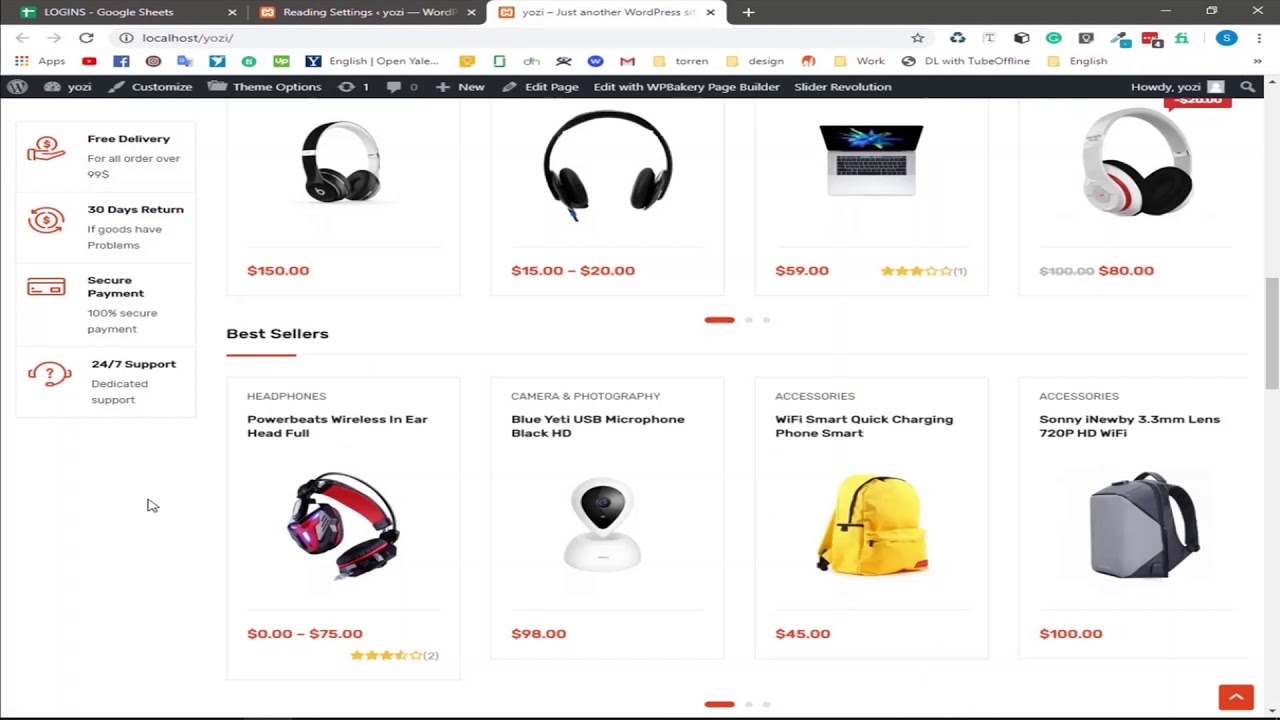The image depicts a user viewing a shopping site on their computer screen. At the top, there are three browser tabs open: "Logins-GoogleSheets," "Reading Settings, Yozi-Word something," and "Yozi-JustanotherWordPress," alongside a plus sign for opening new tabs. Below the tabs is the browser's address bar, displaying the URL "localhost/Yozi/" with standard navigation icons such as back, forward, reload, and a star icon to bookmark the page. To the right, there are multiple icons including a recycling bin, a text editor, a cube, a circled 'G', a gray square, an eyedropper, three red dots, an 'FI' icon, and a user profile image represented by an 'S'. 

The browser interface also shows shortcut icons for various apps like YouTube and Facebook. Below the address bar, there are WordPress-related elements, displaying Yozi's customization options, a "Steam" option, reload icon, comments (speech bubble) icon, a plus sign for adding new items, and edit options for the WPBakery Page Builder and Slider Revolution. There is also a "Howdy Yozi" greeting.

The central part of the screen features the actual shopping site with a white background, touting offers such as "Free Delivery" with a hand holding a coin icon, "30 Days Return" with a circular arrow, "Secure Payment" with a credit card icon, and "24/7 Support" with a headphones icon. Displayed prominently are various products on sale:

- Black headphones priced at $150.
- Another pair of headphones ranging from $15 to $20.
- A laptop priced at $59 with a 3-star rating.
- White headphones priced at $80.
- Red, gaming-style headphones listed between $0 and $75, labeled as "Powerbeats Wireless In-ear Headphone, Best Sellers."
- A section for "Camera and Photography" featuring a Blue Yeti USB Microphone (black) and a white desk microphone priced at $98.
- Accessories like a yellow backpack, a Wi-Fi smart quick charging phone priced at $45, and a futuristic-looking gray backpack.
- The "Sunny iNewbie" 3.3mm lens with 720p HD Wi-Fi capability.

The detailed elements of this image offer a comprehensive view of the products and features available on this shopping site.